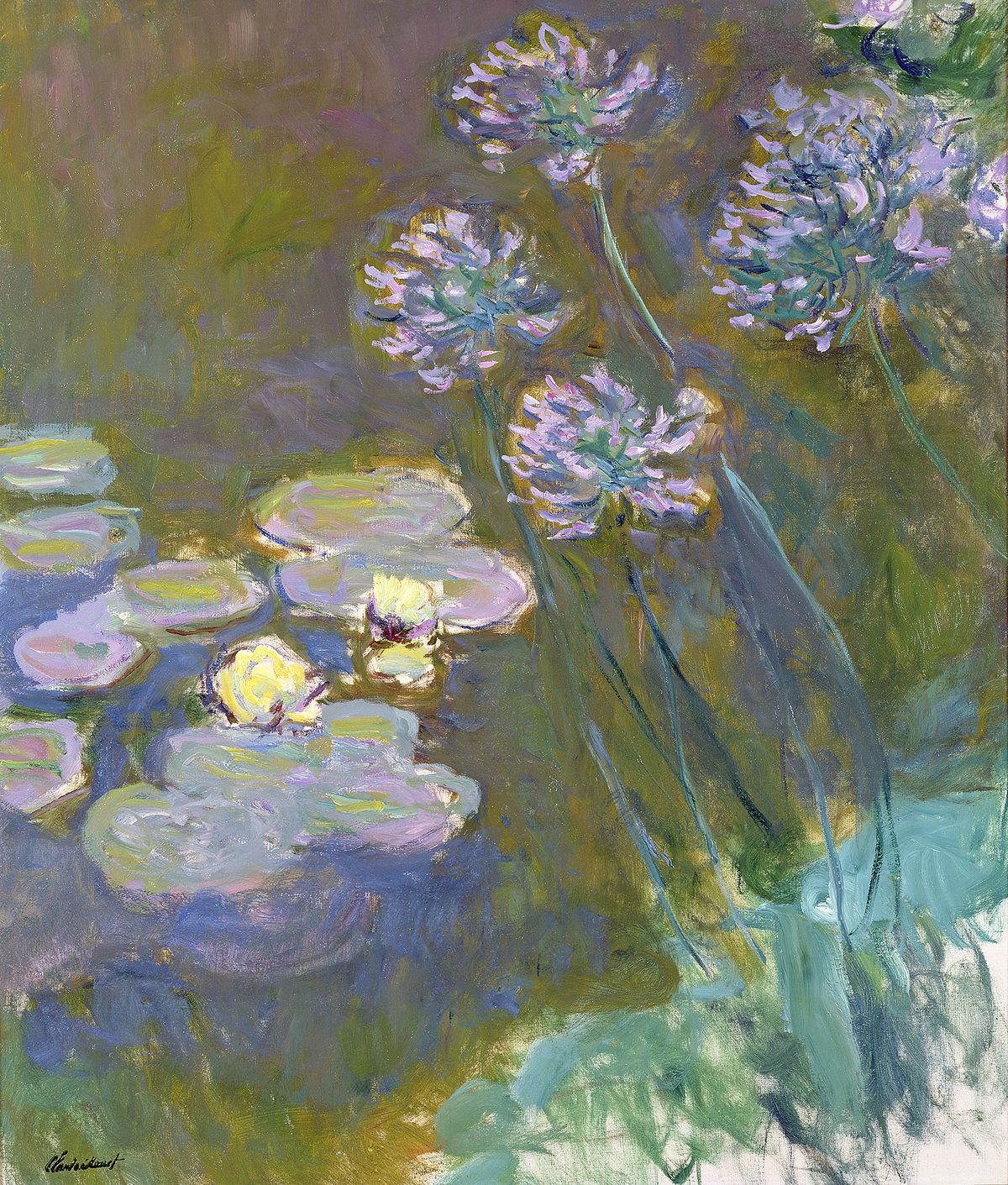This impressionist painting, created by Claude Monet and titled "Water Lilies," features a mesmerizing water scene with a blend of intricate details and subtle color variations. The canvas prominently showcases lily pads and water lilies floating serenely on the surface, which ranges in color from deep green to dark blue, interspersed with muddled patches of brown and reddish-yellow shades. In the top right quadrant, several round, globe-shaped purple flowers with delicate blossoms emerge from long green stems, rooted in the shoreline. Additionally, the bottom right corner highlights a green mass representing the shore. Monet's characteristic black signature can be seen in the bottom left corner. The artwork, a vertical rectangle approximately one and a half times taller than it is wide, masterfully merges shades of pink, purple, green, light blue, and gray, creating a tranquil yet vibrant depiction of a natural water landscape.